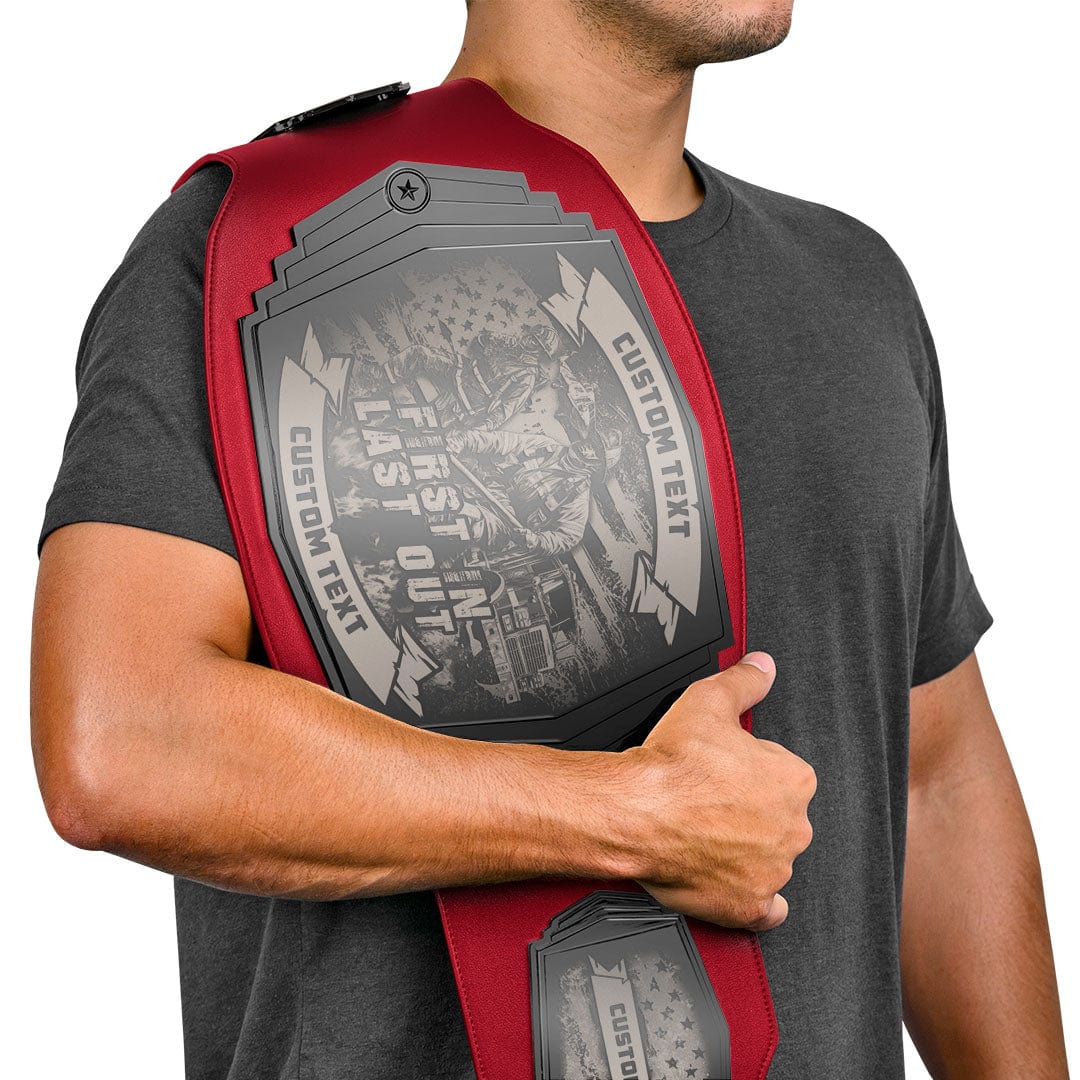In this photograph taken against a white backdrop, we see the upper body of a man with light brown skin wearing a gray, half-sleeve t-shirt. The man's face is partially visible, showing his chin and a hint of black stubble. Draped over his shoulder is a large, red championship-style belt reminiscent of those awarded to professional wrestlers. The belt features a prominent metal face plate in the center, with intricate custom artwork rendered entirely in various shades of gray. This artwork includes a depiction of two firefighters standing in front of a fire truck and an American flag. The belt bears the text "Custom Text" at the top and bottom and "First In, Last Out" in the center. Additionally, there is another smaller face plate on the belt showcasing an American flag print with the word "Custom" inscribed over it.